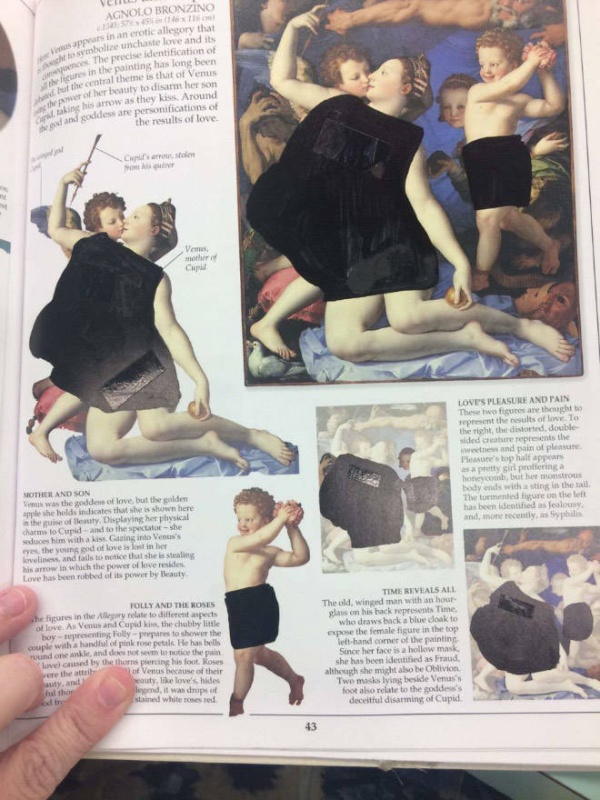The image depicts an open page of a book, likely an art book, with text and artworks on it. The lower left corner of the image shows three fingers holding the page. At the top right corner of the page is a colored oil painting by Agnolo Bronzino, portraying a woman whose nudity is obscured by black ink, along with several children around her. The painting is an old one, possibly from around 1343, and appears to be a religious piece. The page also features detailed photographs and close-up views of different sections of the painting, including a mother holding a staff and her child. Text blocks in black font provide descriptions and contextual information, mentioning phrases such as "love's pleasure and pain" and "time reveals mother and son crawling in the roses." The artworks include medieval representations, such as dancing cherubs and various figures, possibly indicating an array of themes from innocence to maternal care. The page number 43 is visible at the bottom, anchoring the context within the book.